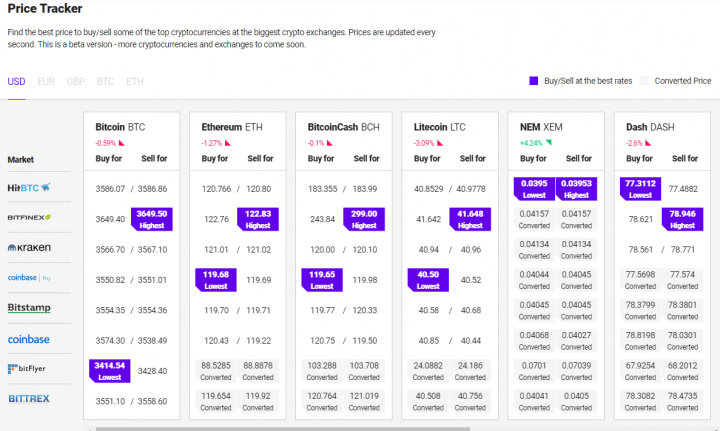The image depicts a user interface of a cryptocurrency price tracking website with a predominantly white or light gray background. In the top left corner, the website header reads "Price Tracker" in bold, black letters. Below the header, a subtext states, "Find the best price to buy/sell some of the top cryptocurrencies at the biggest crypto exchanges. Prices are updated every second. This is a beta version. More cryptocurrencies and exchanges to come soon."

A light gray rectangle occupies the majority of the lower portion of the screen. In the top left of this rectangle, several currency options are displayed, including USD, EUR, GBP, BTC, and ETH, with USD highlighted in purple.

The left column lists various cryptocurrency exchanges: Market, HitBTC, Bitfinex, Kraken, Coinbase, Bitstamp, Bitflyer, and Bittrex. Adjacent to this column are six vertical white rectangles, each providing statistical data and historical value trends for different cryptocurrencies. From left to right, these segments represent Bitcoin (BTC), Ethereum (ETH), Bitcoin Cash (BCH), Litecoin (LTC), NEM (XEM), and Dash (DASH). All cryptocurrencies except NEM (XEM) display red downward arrows, indicating a decrease, while NEM (XEM) shows an upward trend of 4.24%.

In the top right corner of the gray rectangle, a purple square button labeled "Buy/Sell at the Best Rates" is positioned. Adjacent to it, a white square reads "Converted Price."